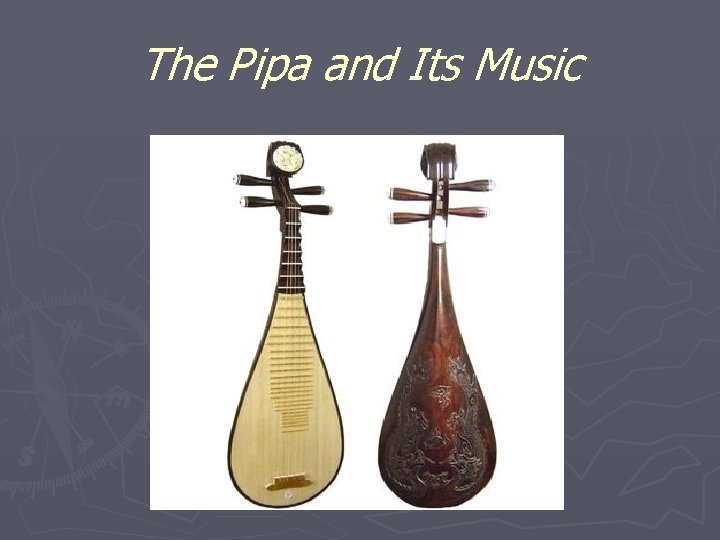The image showcases a detailed poster titled "The Pipa and its Music" in creamy white text against a grey background with light grey lines, some of which converge into a compass design at the bottom left corner. Central to the poster is a white-bordered box featuring two illustrations of the Pipa, a traditional stringed instrument. One side displays the instrument's front, which is crafted from light-colored wood, likely maple, and possesses a dark wood upper section. The Pipa features an oblong, teardrop-like base with four strings running from the top to the bottom, passing over five frets. The headstock is black and adorned with four tuning pegs, which are pieces of wood designed to adjust the string tension. The back side of the Pipa is showcased next to the front, revealing an intricate, ornate design with floral and dragon carvings in dark red wood. The detailed carvings and overall craftsmanship highlight the beauty and complexity of this traditional instrument.